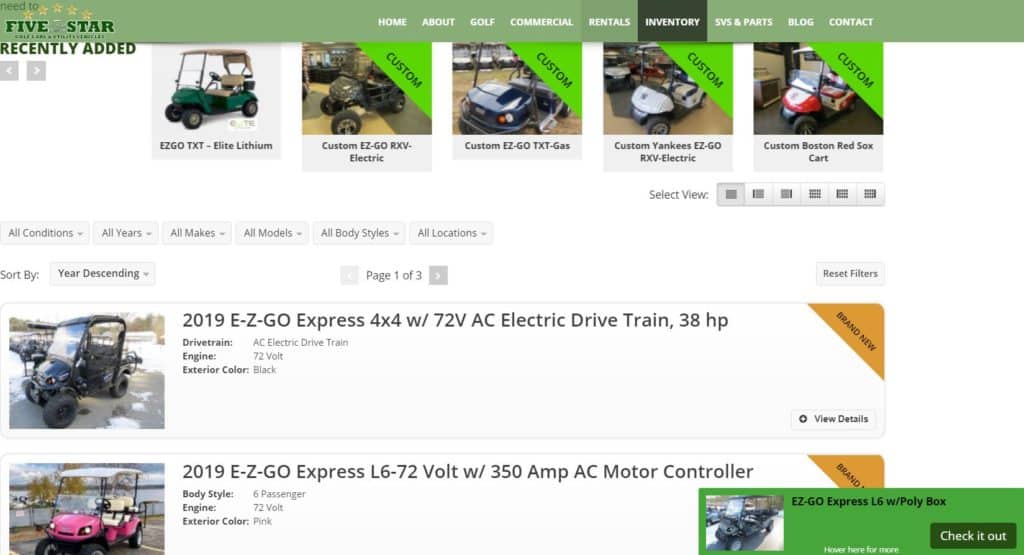The image displays a shopping webpage dedicated to a variety of vehicles, prominently featuring tractors and specialized carts. On the top left corner, there is a "5 Stars" rating icon accompanied by the note "Recently Added." Below this, several vehicles are listed with their respective names: EZgo TXT, Elith Lithium, Custom EZgo RXV Electric, Custom EZgo TXT Gas, Custom Yankees EZgo RXV Electric, and Custom Boston Red Sox Cart. 

To refine the search, a series of categories or filters are provided, including options for "All Conditions," "All Years," "All Makes," "All Models," "All Body Types," and "All Locations." The first vehicle on the page is detailed as a "2019 EZgo Express 4X4," featuring a 72V AC electric drivetrain.